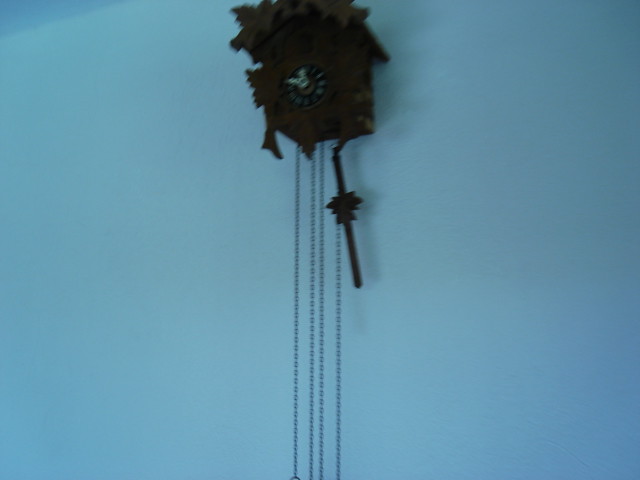This image depicts a wooden cuckoo clock with a dark finish, hanging on a sky-blue wall, though the lighting gives it a slightly different hue. The top portion of the clock's pointed roof is cut off in the frame. The clock, designed in a rectangular shape and resembling a small house, features ornate carvings, including detailed leaves and bird motifs along the top and bottom. Centered in the clock is a black face with white hands and numbering, showing the time at 11:50. Below the clock face, four dark chains hang straight down, though their endpoints are not visible. Additional carved details, including a lever with a carved element skewing to the right, dangle from the clock's base.